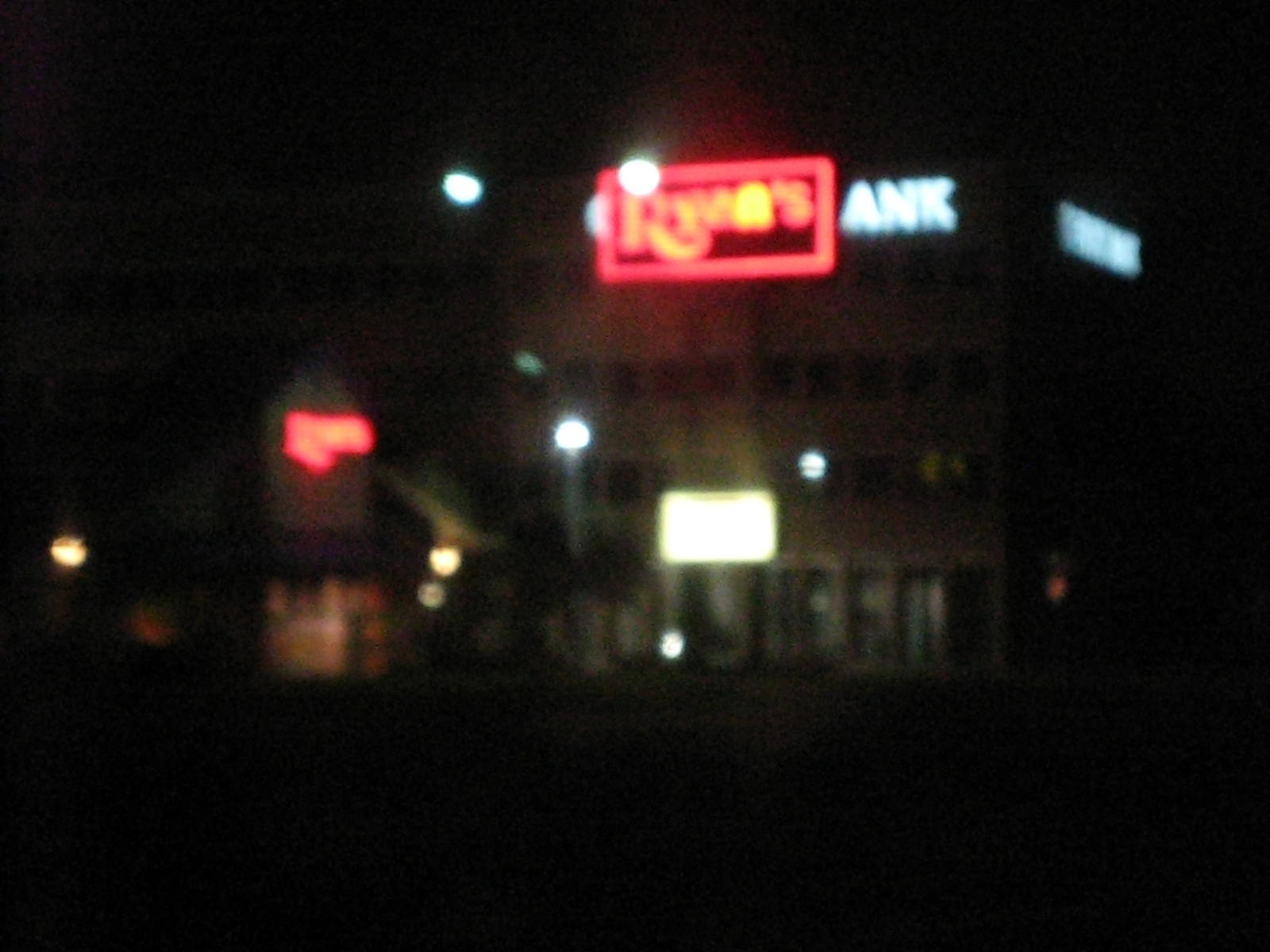A blurry nighttime photograph of a bustling commercial area featuring various illuminated stores and shops. The focal point is a two- or three-story building centrally located in the otherwise dark image. At the top of this building, a red neon-lined rectangular sign with indistinct yellow writing stands out. To the top left of this sign, two round white shapes are visible. On the right side of the red-outlined sign, the letters 'A' and 'N' are illuminated in white. Continuing around the corner of the building to the right, there appears to be additional white lights. The ground level of the building showcases a series of plate glass windows or doors, with a glowing rectangular white light above the central entrance. On the left side of the image, numerous yellow and white lights dot the scene. In the foreground, there is a diagonally positioned lower storefront adorned with bright red neon lines and a red sign perched atop it.